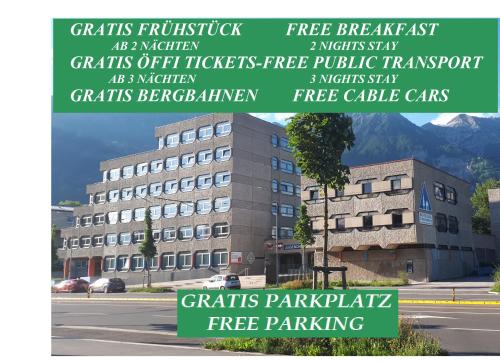The advertisement depicts a striking multi-layered, pyramid-shaped hotel building crafted from gray stone. The structure features uniform windows and a small red entrance to the far left. Set against a backdrop of majestic mountains, the building is surrounded by lush green grass and a tree, with a road running in front. A green banner at the top, with text in both German and English, details enticing amenities: "free breakfast with a two-night stay," "free public transport with a three-night stay," and "free cable cars." A thinner green banner at the bottom also indicates "free parking" in white text. The polished brutalist architecture and serene landscape evoke a sense of modern luxury amidst natural beauty.